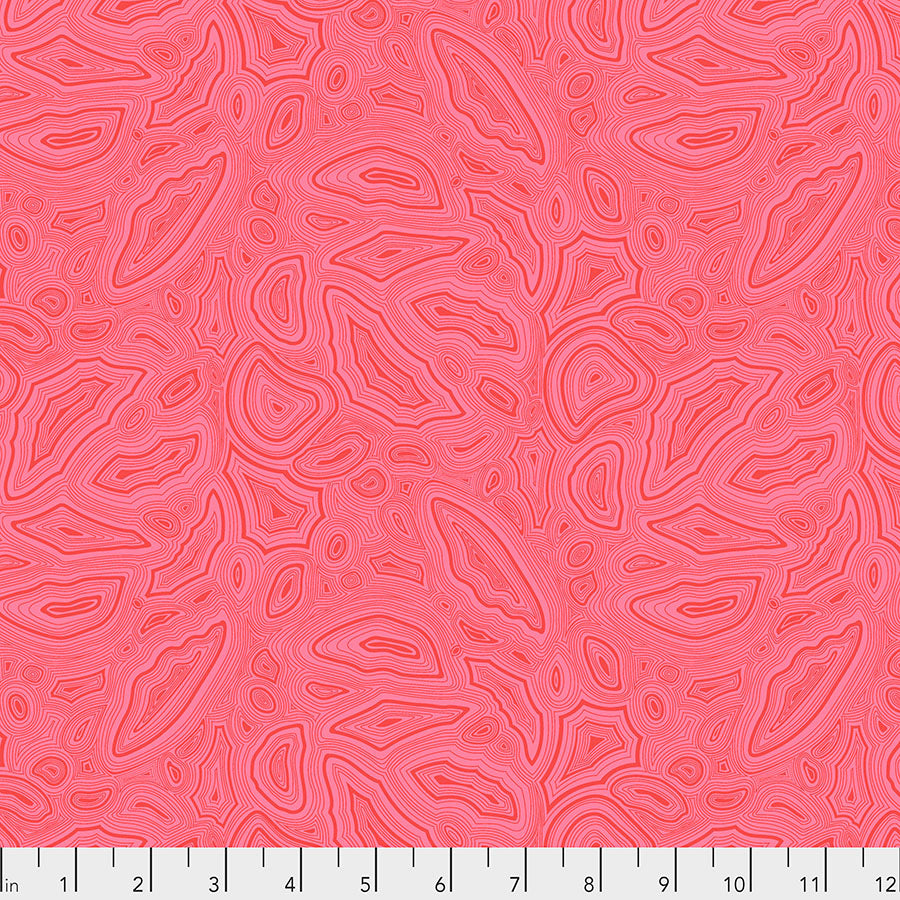The image features an intricate line drawing that resembles the inside of a geode, characterized by organic, concentric shapes with various hues of pink, from light to a darker, almost orangish pink. These rings and shapes intertwine and merge, creating an abstract, textured pattern that evokes the natural layers found in semi-precious stones. The bottom of the image includes a white ruler marked in black from 0 to 12 inches, with finer black lines denoting the half-inch increments. The overall effect is a striking blend of geological precision and abstract art, meticulously measured and presented.